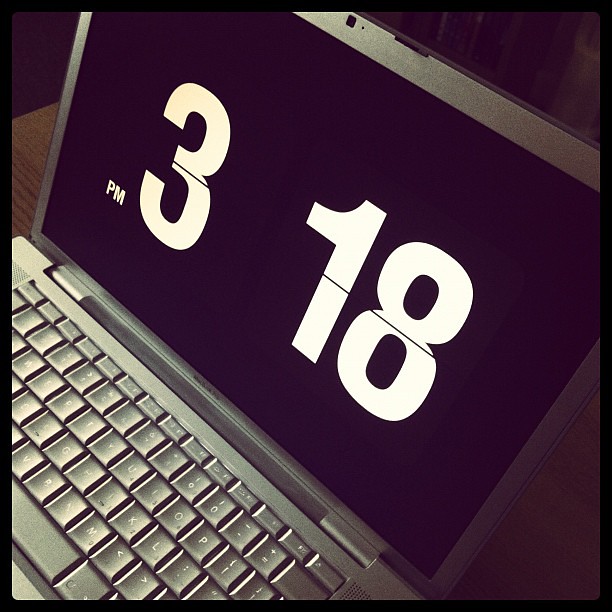The image is a photograph of a grey laptop, viewed from a slightly sideways angle, resting on a brown wooden surface. The screen, with a black background, prominently displays the time as "3:18 PM" in large, white numbers. There is a noticeable gap between "3" and "18," and a horizontal black line bisects the screen, mimicking the style of old fashioned flip clocks. The laptop's keyboard is visible beneath the screen, with a small webcam at the top of the display. The overall aesthetic of the photograph is modern, with shading and perhaps a subtle filter that adds a bit of a sepia tone. The details make it hard to discern whether the image is a real photograph or a digitally created graphic.